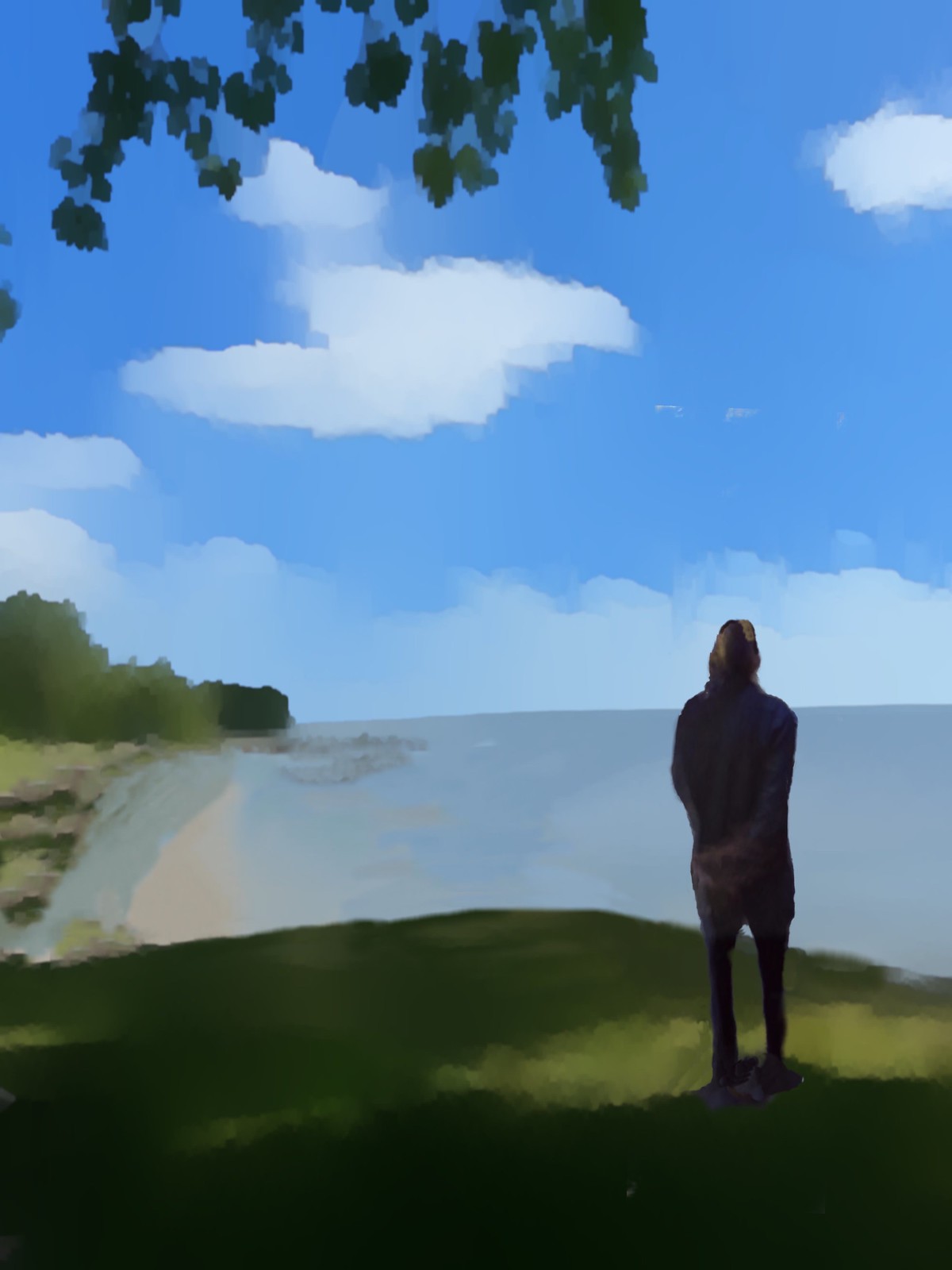In this landscape painting, the foreground features a lush expanse of green grass that flows from the left side of the frame and curves slightly outward before tapering back in on the right. At the bottom center of the image, the rough sketch of a figure with their back to the viewer can be seen. The person is dressed in black leggings and a long, mid-thigh-length sweater, with their blonde hair cascading down their back and one arm tucked behind them. They appear to be contemplatively gazing out over a serene body of water.

To the left, a small strip of land extends into the water, leading to a cluster of trees. The sky above is a rich blue, dotted with several fluffy white clouds. In the upper portion of the painting, branches from an overhanging tree frame the scene, their green leaves adding to the composition's sense of tranquility and natural beauty.